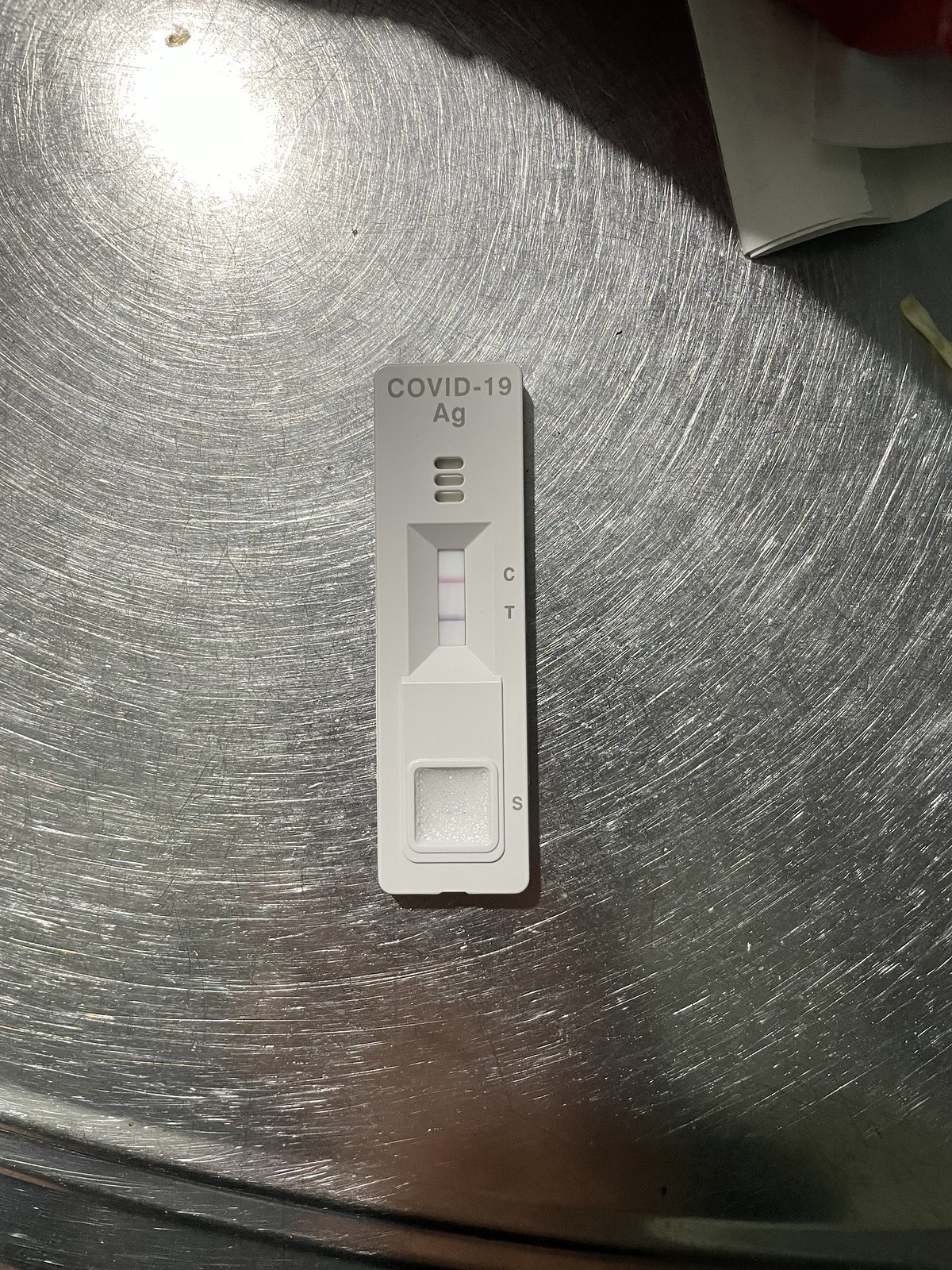This top-down image captures a COVID-19 antigen test kit placed on a metallic, machine-finished surface. The surface reflects a bright light in the upper left-hand corner, while the upper right corner is cast in shadow. Within this shadow, partially visible items include a napkin, a small stick, and the red edge of what appears to be a cup.

The test kit itself is made of white plastic, designed in a rectangular shape. At the very top of the kit, "COVID-19 AG" is printed in gray. Below this text are three gray oval shapes. Further down, there is a rectangular white box displaying two colored lines; the top line is red, indicating the control line (C), and the bottom line is blue, denoting the test line (T). To the right of these lines, the letters "C" and "T" are written in gray. At the bottom of the kit, another white square is labeled with an "S" in gray. The meticulous details and the stark contrast of light and shadow provide a clinical yet vivid portrayal of the test kit and its surrounding environment.